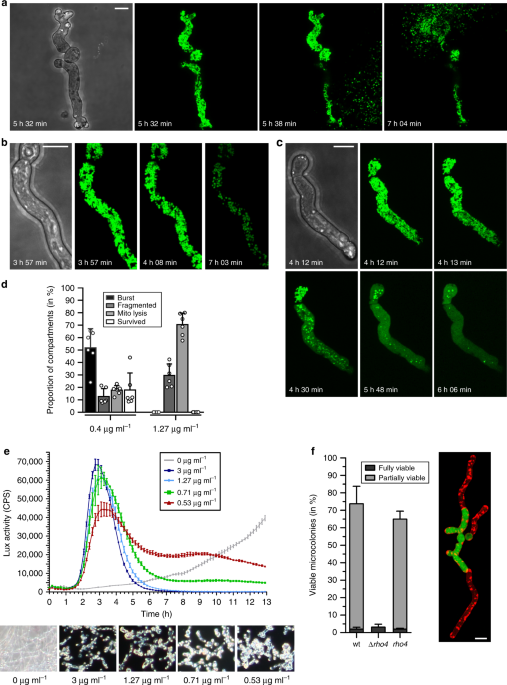The vertically rectangular, multi-color composite image is made up of numerous smaller images and charts, set against a primarily white background with no definitive border. The layout is divided into sections labeled A through F, featuring various microscopic black and white images, some highlighted in neon green, illustrating microorganisms. The top parts of these panels showcase complicated graphs, measuring in nanograms per milliliter, with values ranging from 0, 0.53, 0.71, 1.27, to 3, depicted in intricate detail. There are numerous bar and line graphs scattered across the image, predominantly situated in the central and lower sections. The line graphs use red, green, and blue colors. Additionally, black rectangles with glowing green streaks and dark gray rectangles with outlined streaks are also visible, showcasing microorganisms under a microscope. In the bottom left corner, black and white photographs are present, while a mix of multi-colored pictures and further charts reside on the right side. Text conveying time in hours and minutes is also embedded within the image, adding to its detailed complexity.